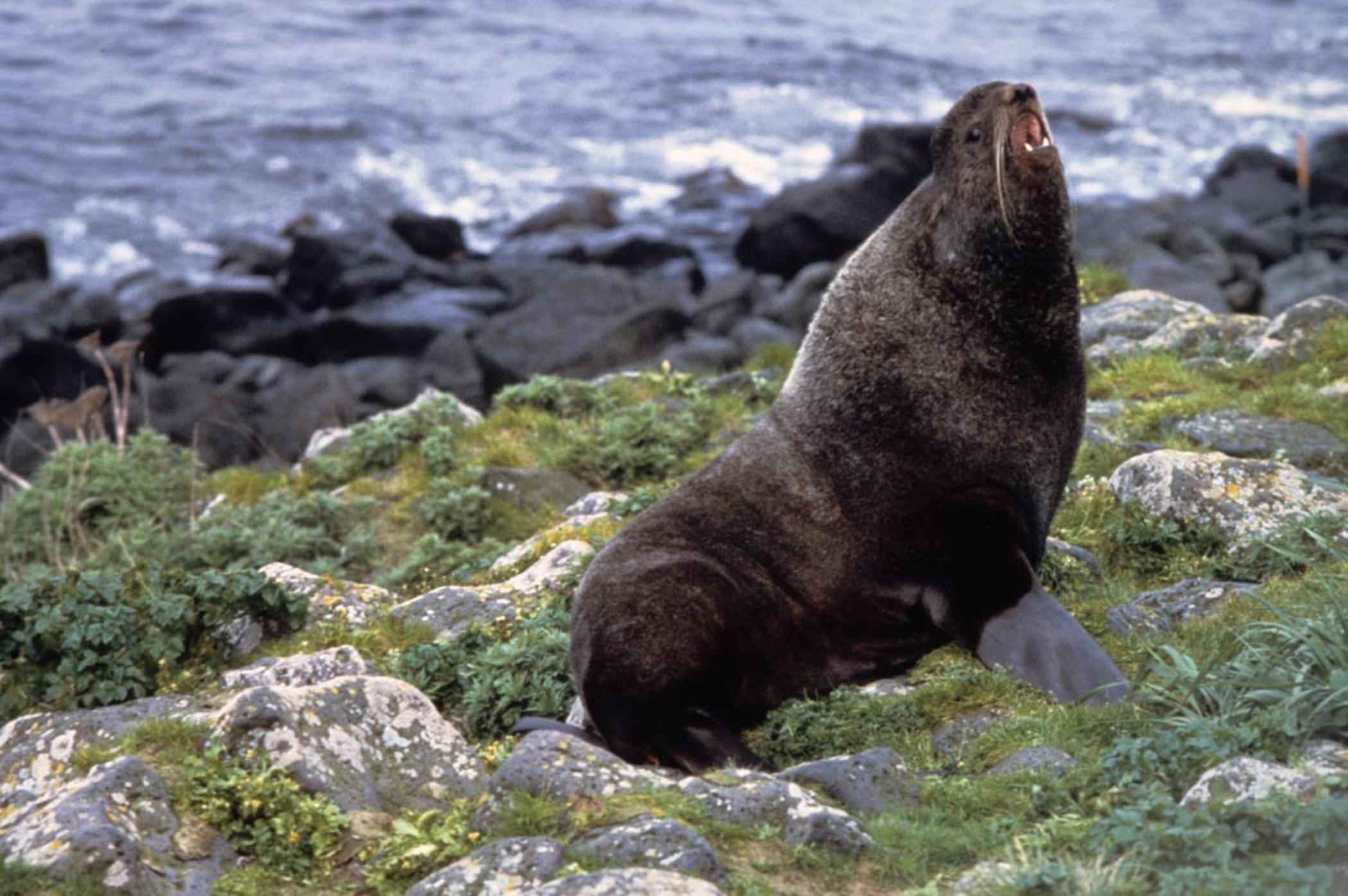The image depicts a large marine mammal, possibly a sea lion or walrus, though it lacks tusks, situated prominently on coastal rocks. The creature, characterized by its dark brown, short, thick hair and black flippers, is positioned towards the middle right of the photograph, facing upwards with its head tilted back, mouth open as if calling out, displaying two small white teeth and long whiskers drooping down from its nose. Its black eye gazes slightly off-center, adding a lifelike touch. The animal's upright posture shows its front flippers planted firmly on the rocks, while the back flippers rest on the ground.

The surrounding environment features wet, jagged rocks interspersed with patches of light and dark green vegetation, along with some white markings. Further in the background, the rocky coastline continues, fading into a dark, gray-blue ocean with white foam where waves break against the shore. The setting is an outdoor, daylight scene, emphasizing both the rugged textures of the coastal landscape and the natural colors of the sea and flora.